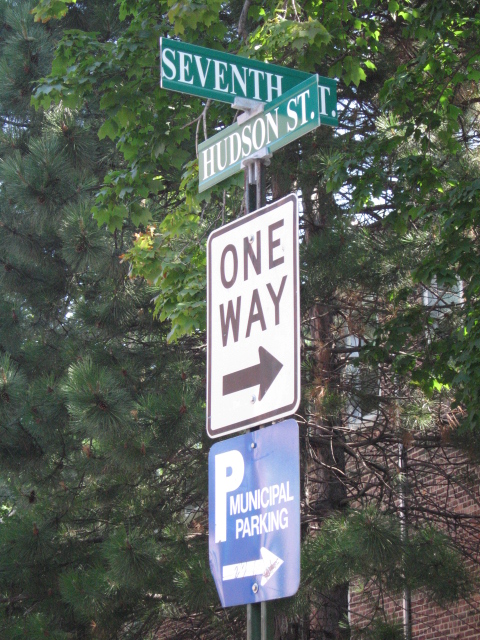This image captures an intersection marked by several street signs. Towering above, at the top of the signpost, is a hunter green 7th Street sign, immediately followed by another for Hudson Street, indicating the confluence of these two streets. Below them, a white One Way sign with black letters and an arrow directs traffic to the right. Further down is a blue Municipal Parking sign, which is dented and dirty, adorned with white lettering and an arrow, also pointing to the right. The signpost itself stands in front of a backdrop featuring a red brick building with a lighter-colored roof, its windows framed in white. The greenery surrounding the scene includes both cedar and regular trees, with evidence of the seasonal change in the form of a yellow leaf. The sun brightens the setting, casting light on the leaves clinging to the branches. The entire scene suggests a residential or mixed-use area, with a hint of fall in the air.